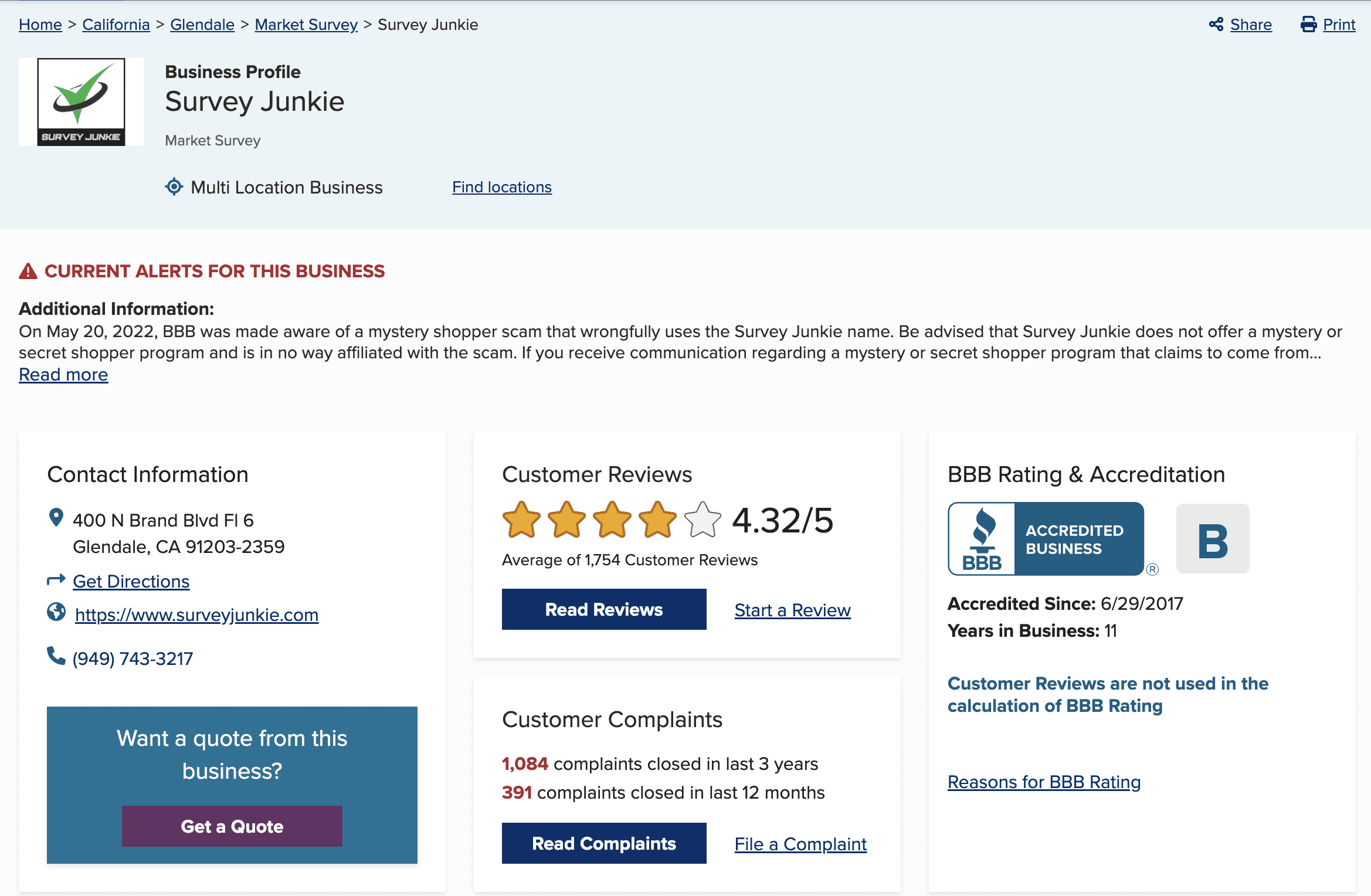Survey Junkie Details and Alert: California Business Profile

**Business Name:** Survey Junkie
**Location:** Multi-location business headquartered at 400 North Brand Boulevard, Floor 6, California.

**Accreditation:** Accredited by BBB since June 29, 2017.
**Years in Business:** 17 years.

**Customer Reviews and Ratings:**
- **BBB Rating:** Not calculated using customer reviews.
- **Overall Rating:** 4.32 out of 5 stars, based on 1,754 customer reviews.
- **Breakdown:** Four gold stars and one silver star.
- **Customer Complaints:** 
  - 1,084 complaints closed in the last three years.
  - 391 complaints closed in the last 12 months.

**Important Alert (May 20, 2022):**
The Better Business Bureau (BBB) became aware of a mystery shopper scam misusing Survey Junkie's name. Survey Junkie does not offer any mystery or secret shopper program and has no affiliation with this scam. If you receive any communication about such a program supposedly from Survey Junkie, it is fraudulent.

For more information, to read customer reviews, file a complaint, or get a quote, please visit the BBB’s business profile page for Survey Junkie.